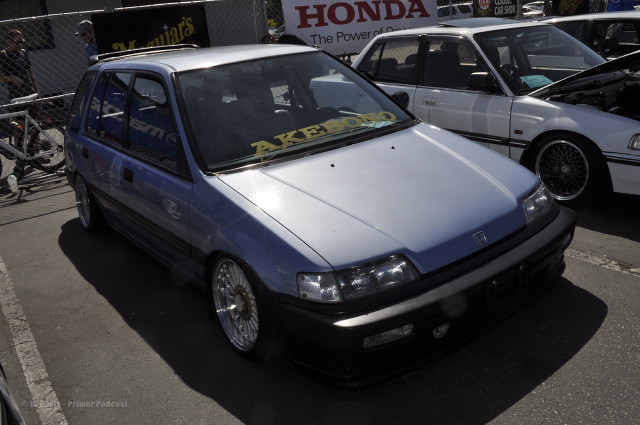In a parking lot with faded white lines and asphalt, a detailed scene centers on a prominently displayed light blue Honda, adorned with chrome spike wheels. The car, a souped-up, custom model that looks like a wagon or sedan from the 80s or 90s, features a notable Akebono decal in gold letters on the front windshield. Parked in front of a chain-link fence, the area behind the car includes visible bicycles and signage for both Honda and Meguiars, suggesting an automotive-themed event or display. To the right of the blue Honda is a white boxy sedan with its hood lifted, displaying a green piece of paper in the windshield and marked with a "Honda, the power of dreams" sign attached to the fence. Another partial glimpse of a white vehicle roof can be seen further right. The lower left corner of the image includes a "Primer Podcast" mark, enhancing the scene's automotive culture ambiance.